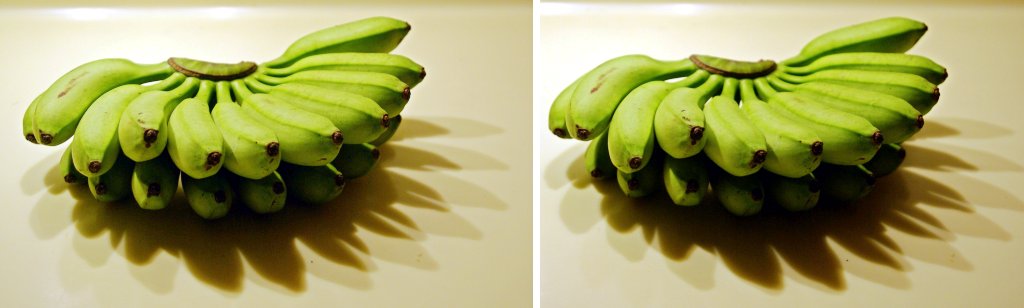This image features two nearly identical, well-lit photos of the same bunches of natural, unripe green bananas. Each bunch is quite large, containing at least 16 bananas, with short, clustered fruits that would more likely be grown in a backyard rather than purchased from a grocery store. The bananas in both photos are positioned on a light brown table, arranged in two rows stacked on top of each other in a fan-like shape that resembles a hand fan or Japanese fan. The bananas have brown tips and a brown stem section at the top, with a distinct shadow cast in front of them, creating a spiky, floral pattern on the table due to the backlighting from a light source located to the upper far left. The photo on the right is slightly lighter than the one on the left, displaying nuanced differences in lighting conditions but otherwise remaining identical.